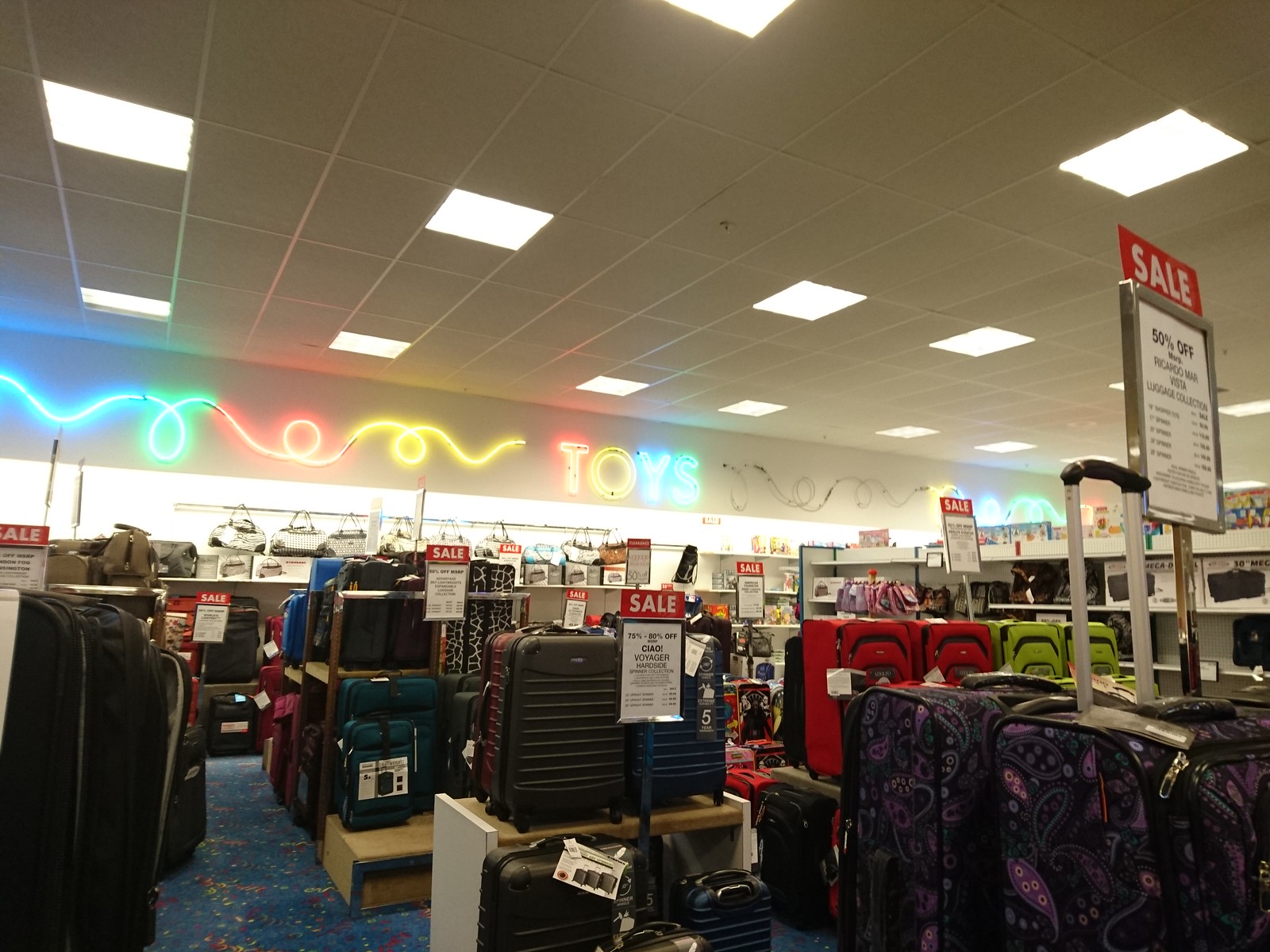A detailed photograph captures the luggage section of a store reminiscent of TJ Maxx or Marshalls. Dominating the bottom third of the image is an array of both small and large suitcases positioned on a combination of shelving units and pedestal-style stands. The luggage displays a palette largely consisting of dark hues, interspersed with vibrant splashes of lime green and red located toward the right-center, while black pieces are scattered further back on the left. The store ceiling, visible in the image, is composed of square white tiles, punctuated by periodically positioned smaller squares of lighting fixtures that show up as whiter spots against the slightly off-white backdrop of the ceiling. Centrally featured in the image, running horizontally from left to right with a gentle dip on the right side, is a neon sign. This sign showcases a whimsical, swirly line in blue, green, tan, and yellow, culminating on the right end with the word "Toys" illuminated in neon.